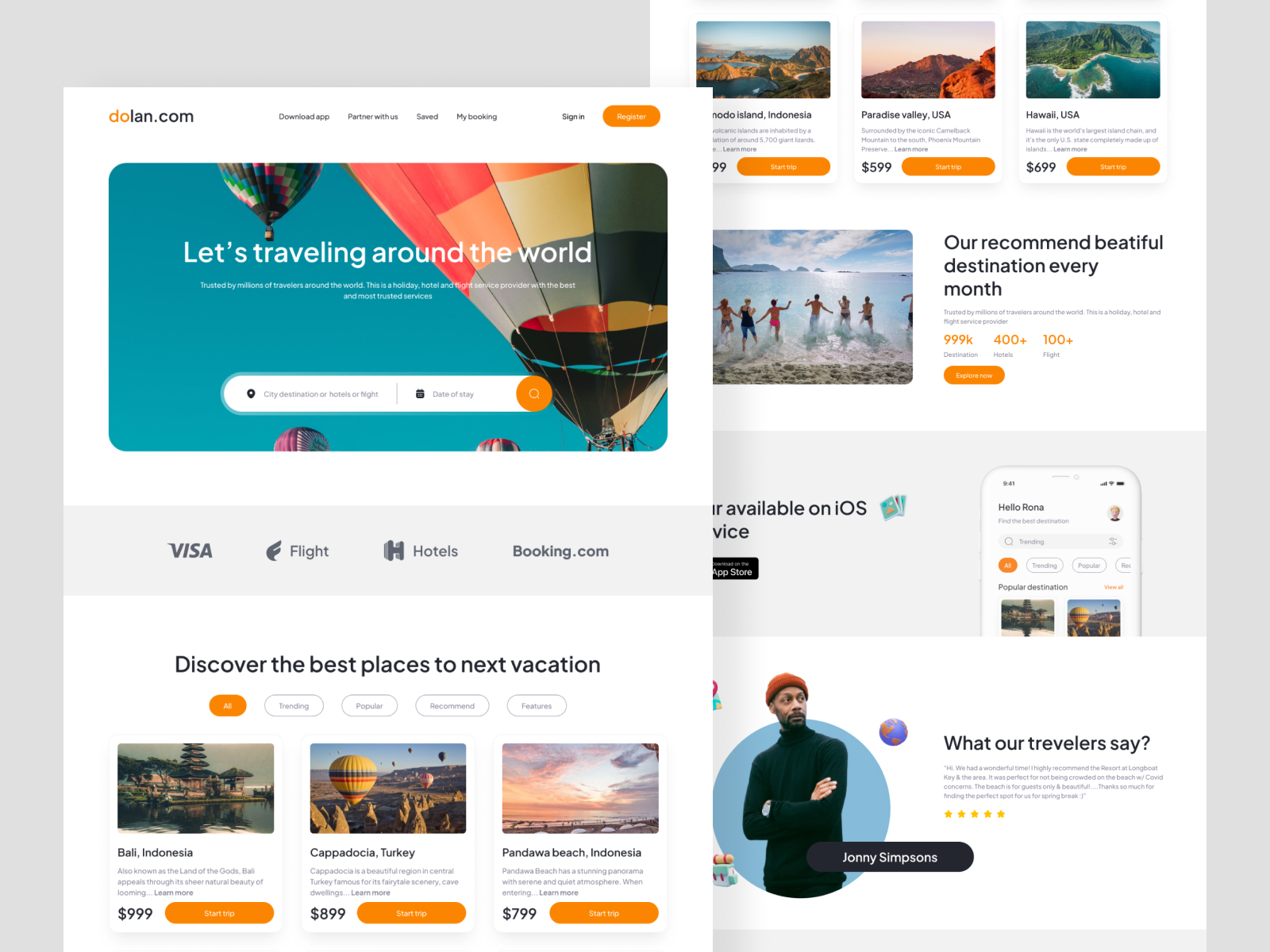In the image, captured as a screenshot, a computer screen displays a website with a grey background. Dominating the screen are two large, overlapping pop-ups, both with white backgrounds that cover almost the entirety of the display.

The first pop-up, positioned at the back, showcases various travel destinations such as Indonesia, Coruscant Valley, and Hawaii. Accompanying these names are scenic photographs portraying mountains and other picturesque views. Each destination includes a price tag, visibly marked as $5.99 and $6.99, with another price partially obscured.

Superimposing this, the second pop-up prominently features the website's name, "dooland.com." Here, 'do' is highlighted in orange, while the rest of the text is in black. This pop-up provides navigational options including "Download App" and "My Bookings," though a few options are truncated and not fully visible. Additionally, there are fields for signing in and registering; the "Register" button is distinctively colored with white text over an orange bar.

The second pop-up bears the motivational tagline, "Let's travel around the world," accompanied by graphics of hot air balloons. Below this, a search bar is present with options labeled "Location," "Visa," "Flight," "Hotels," and a mention of "booking.com." It also invites users to "Discover the best places for your next vacation," featuring destinations such as Bali in Indonesia and Turkey, alongside various travel prices.